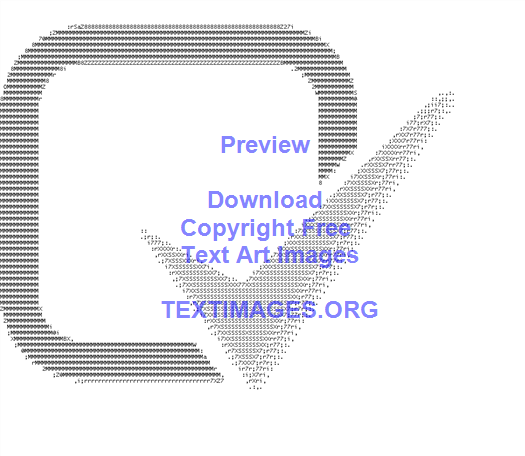The image is an artistic advertisement for textimages.org, showcasing a computer-generated, intricately designed icon. At the center of the image is a rounded square, outlined with closely spaced lines and dashes in mixed shades of blues, grays, and blacks, giving it a dimensional appearance. A lighter-colored checkmark starts from the upper right of the image, extending down and across the right side of the square, with the tip pointing towards its white center.

The text "Preview, Download Copyright-Free Text Art Images" appears prominently in light blue letters against the intricate background, with "textimages.org" below it. The text placement is largely on the right side of the image. This advertisement effectively blends artistic design with informational content, using a combination of dots, dashes, and varied shading to create an eye-catching visual representation.